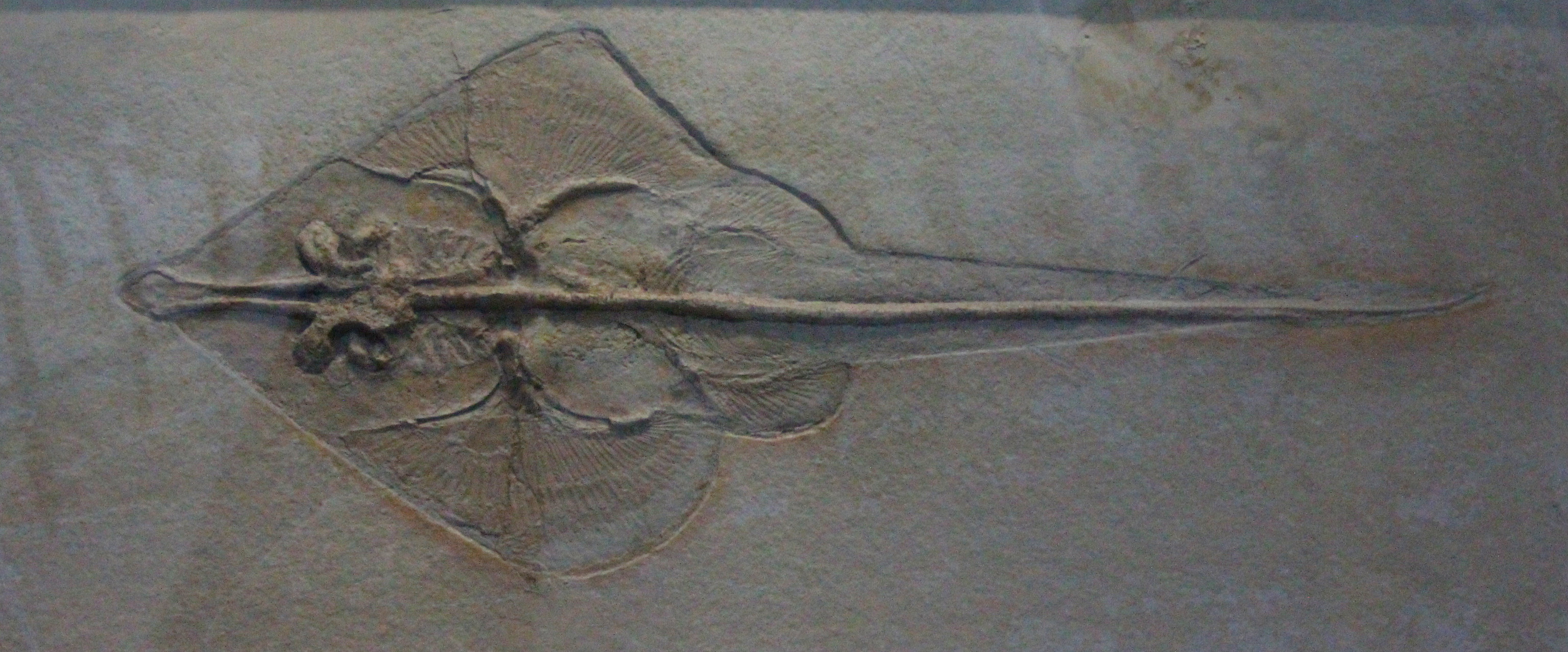This close-up image captures a highly detailed fossil of a stingray, encased in what appears to be a glass enclosure, with noticeable reflections on its surface suggesting an indoor setting, likely a museum. The stingray fossil, positioned horizontally in the center of the image, displays intricate details of its radial lines and fin marks, with its head pointing left and tail extending to the right. The encompassing rock matrix is primarily beige and white, seamlessly blending into the fossil's gray, black, brown, and white hues. The fins stretch almost to the top and bottom edges of the frame, underscoring the fossil's prominent and well-preserved nature within the stone.